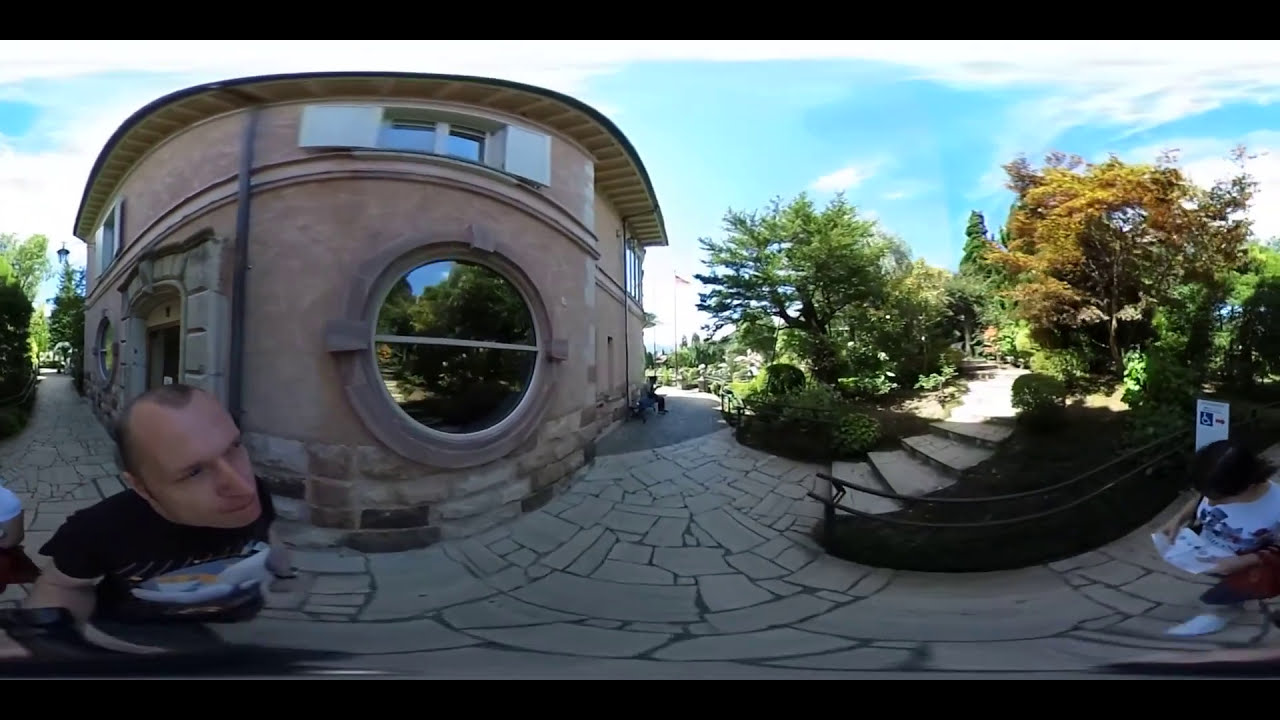The photograph, captured with a fisheye lens, presents a slightly distorted panoramic view of a cobblestone plaza in a city, featuring a tall, historical building with stone siding and smooth plaster in light tan. The building's most striking feature is a giant circular porthole window, reminiscent of a submarine’s design. In the foreground, the cobblestone plaza with irregularly-shaped flat stones stretches across the image, creating an organic pattern with darker edges between the stones. 

To the right, stairs lead up into a lush, woodland path surrounded by dense, leafy trees and bushes. There is also a fence nearby, adding to the natural landscape that juxtaposes the urban setting.

In the bottom left corner, a middle-aged man with balding hair and wearing a black t-shirt with a design is captured. Due to the fisheye effect, his face appears disproportionately large as he looks to the right. He stands out against the meticulously detailed background with a serious expression on his face.

Additionally, there is a woman with dark hair and a white shirt, also looking down at a pamphlet as she walks. A seated person on a bench can be seen near the building, perhaps engaged in reading.

Above, the sky is bright blue with scattered clouds, completing this scene that seamlessly blends historical architecture with the bustling energies and tranquil green spaces of the city.